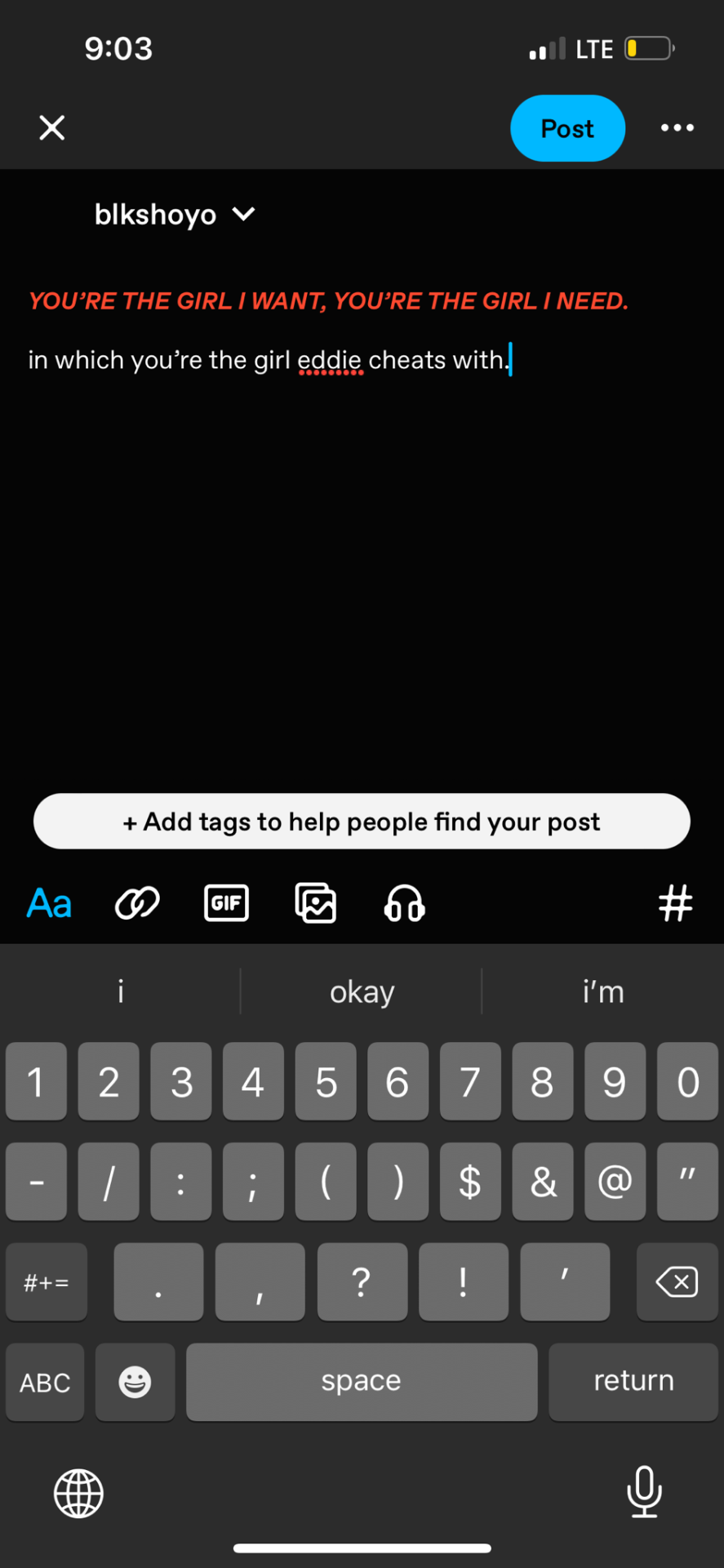The image is a screenshot from a social media or content-sharing platform. The screen displays a status bar at the top with the time reading 9:03, LTE signal strength, and battery status icons. The username "BlackShowYo" is visible at the top, with a dropdown arrow next to it, indicating a menu or additional options.

Below the username, the text being composed in the post is formatted in red, bold, and italic and reads: "You are the girl I want, you are the girl I need. In which years you are the girl Eddie cheats with." The name "Eddie" is underlined with red dots, indicating a possible spelling or grammar error.

The post interface is highlighted in blue, suggesting that the post is in progress. Various interactive elements such as the ability to share opinions, tag people, and add media are visible. There is a keyboard at the bottom of the screen along with a GIF icon, allowing users to insert GIFs into their posts. Overall, the image captures the standard functionalities of a social media posting interface.